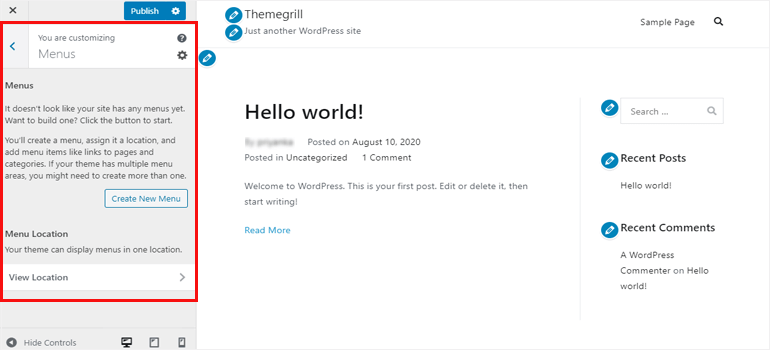This is an intricate screenshot of a WordPress website interface. The overall background of the site is white. On the left-hand side, there's a vertical gray column extending from the top to the bottom. In the upper left corner of this column is a black "X." On the upper right corner of the gray box, there is a blue button labeled "Publish."

Moving downward in the column, a red box features a blue arrow on its left side, accompanied by a white stripe. The section is labeled "You are customizing menus" and includes a question mark and a small star on the right. Below this section, bold black text reads "Menus," followed by a message stating, "It doesn't look like your site has any menus yet. Want to build one? Click the button to start. You'll create a menu, assign it a location, and add menu items like links to pages and categories. If your theme has multiple menu areas, you might want to create more than one." Beneath this message, there's a white button outlined in blue with blue text that says "Create Your Menu."

Further down is another bold black title saying "Menu Location," which explains, "Your theme can display menus in one location." Below it is a white bar with black text saying "Your view location," accompanied by a left-facing arrow. At the very bottom of the gray column, outside the red box, there are options labeled "Hide Controls," which display three different control icons.

In the center of the screenshot, the text "Theme Grill - Just Another WordPress Site" appears with an adjacent blue circle featuring a pencil icon. Also, there's a sample page in the upper right corner paired with a search bar. Centrally positioned, in bold black text, it reads "Hello World!" followed by "Posted on August 10th, 2020" and "Posted in Uncategorized, One Comment." The message continues with "Welcome to WordPress. This is your first post. Edit or delete it, then start writing." Below this message, a blue link labeled "Read More" is visible.

On the right side of the screenshot, a faint white box contains a button and three distinct sections, each marked by a blue circle with a pencil icon. The first section includes a search box, the second section, in bold black text, reads "Recent Posts" with the entry "Hello World" beneath it. The third section, also in bold black, says "Recent Comments" with text under it stating, "A WordPress commenter on Hello World."